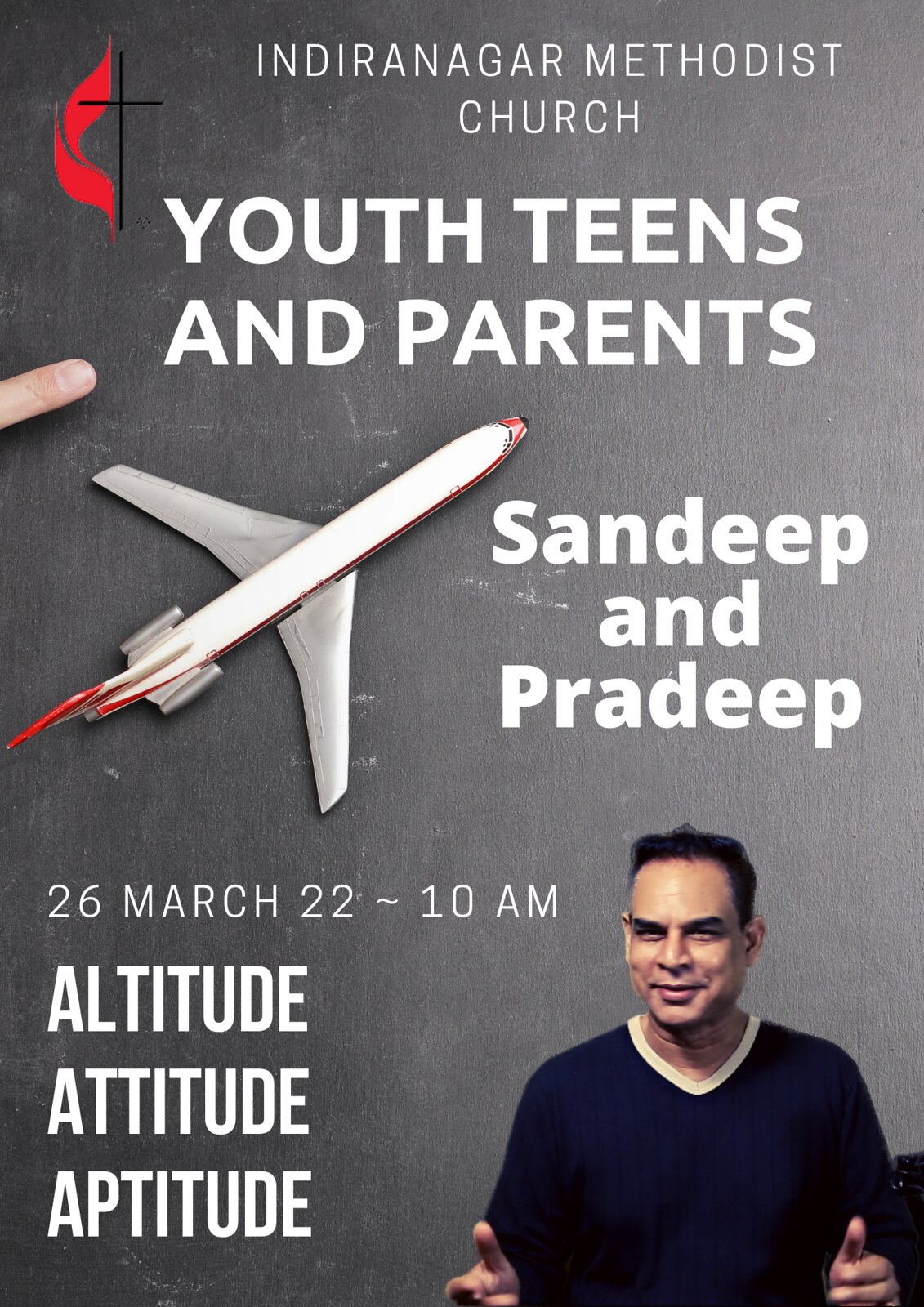The image is a detailed announcement for an event hosted by the Indiranagar Methodist Church, set against a dark gray background. In the upper left corner, there's a logo featuring a cross entwined with a flame, next to which "Indiranagar Methodist Church" is written in a white font. Below this, also in white, the text reads "Youth, Teens and Parents." Centered in the image, there is a prominent, overhead view of a white airplane with red markings on its nose and tail. This section includes "Sandeep and Pradeep" in the middle, indicating the speakers or hosts of the event. The lower part of the image displays further details: on the left, it lists the date and time "26 March 2022 at 10 a.m.," and beneath that, the words "Altitude, Attitude and Aptitude" are prominently featured. In the bottom right corner, there's a photograph of an Indian man, likely one of the speakers Sandeep or Pradeep, who is dressed in a black v-neck shirt with a white collar. He has dark hair and a cheerful expression. The man appears to be giving a thumbs-up gesture, reinforcing the inviting and motivational tone of the announcement.